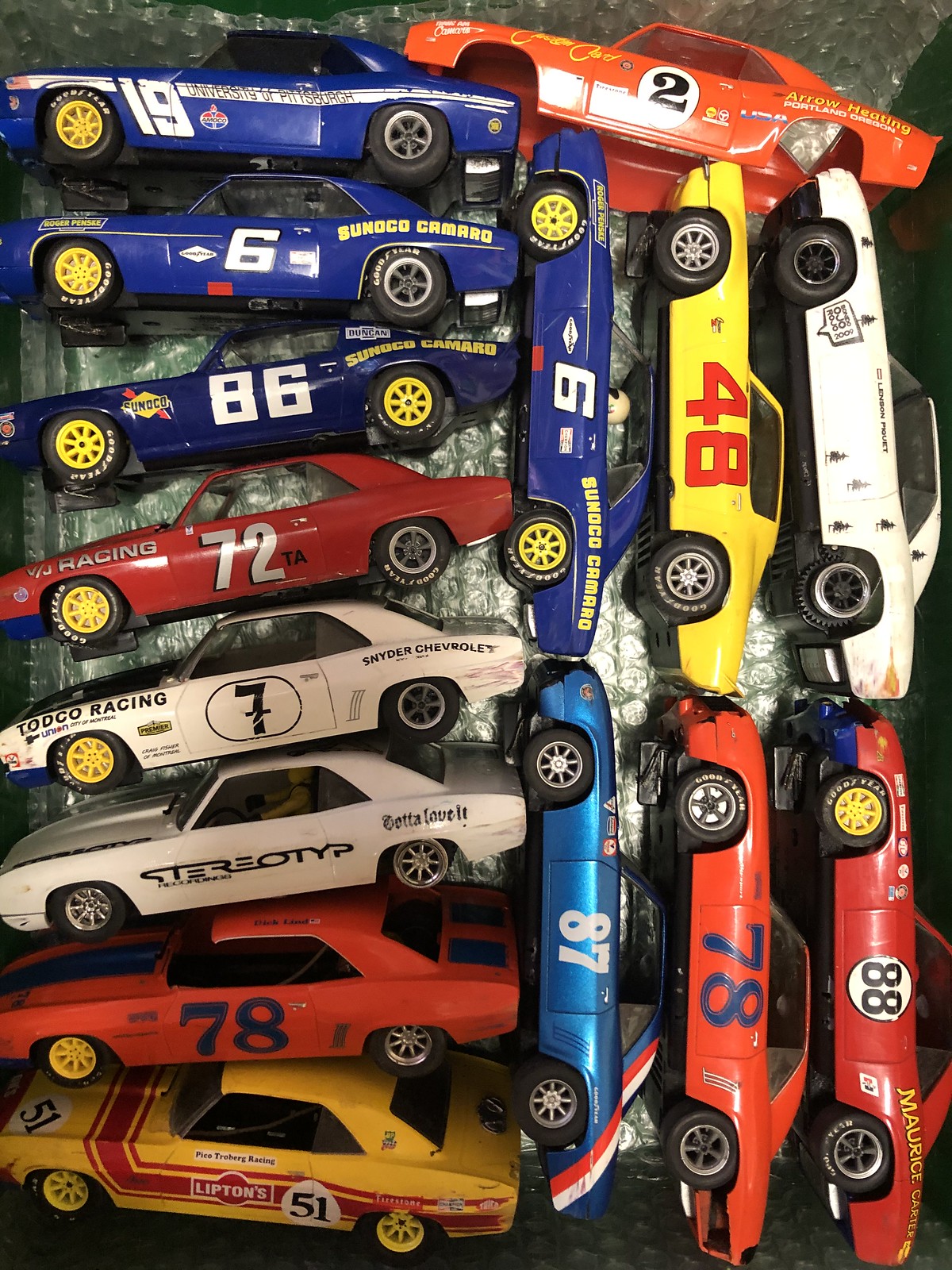This is an overhead photograph of a collection of model racing cars, reminiscent of Hot Wheels, organized in two distinct arrangements. On the left side, nine cars are stacked horizontally on top of each other. Starting from the top, there are four blue cars, identified by numbers such as 6 and 86, followed by a red car with the number 72, two white cars where one displays the number 7 and the other has no number, an orange car with 78, and a yellow car marked 51. Each car is adorned with various sponsor logos, highlighting their racing theme, and they all feature black wheels with yellow centers. On the right side, two columns of three vertically-stacked cars are visible. The colors and numbers of these cars include a blue car with the number 6, a yellow car with the number 48 in red, a white car without a number, a blue car with 87, an orange car with 78, and a red car marked 88. At the very top of these vertical stacks lies the shell of an orange car. The varied colors and numbered liveries suggest these model cars are from a different era, likely the 70s, adding a nostalgic touch to the collection. Together, there appear to be at least fifteen cars in the image.